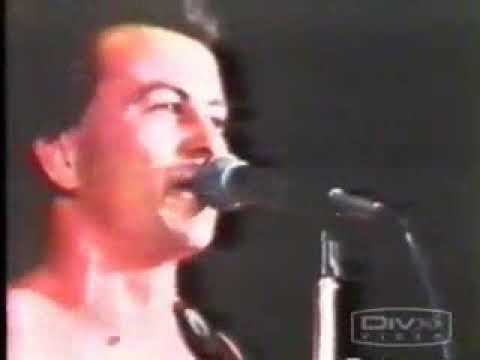This image captures a band performing live on stage, set against a predominantly dark background with teal accents on the left. The focal point is a man playing a beige guitar on the left side of the stage, dressed in a light pink or beige shirt. His facial expression seems disengaged or frozen. To his left, there's a blue amplifier or station with a silver keyboard or MIDI machine on top of it. The right side of the image features a drummer wearing a black shirt, playing black or silver drums. A stand-up microphone is visible near both performers. The bottom right corner of the image is marked with a white-bordered logo that reads "DIVX" and below it, the word "VIBE". Additionally, there is text across the screen that includes the words "CITY" and "LIVE". The overall atmosphere suggests an indoor concert setting with a dim, moody ambiance.